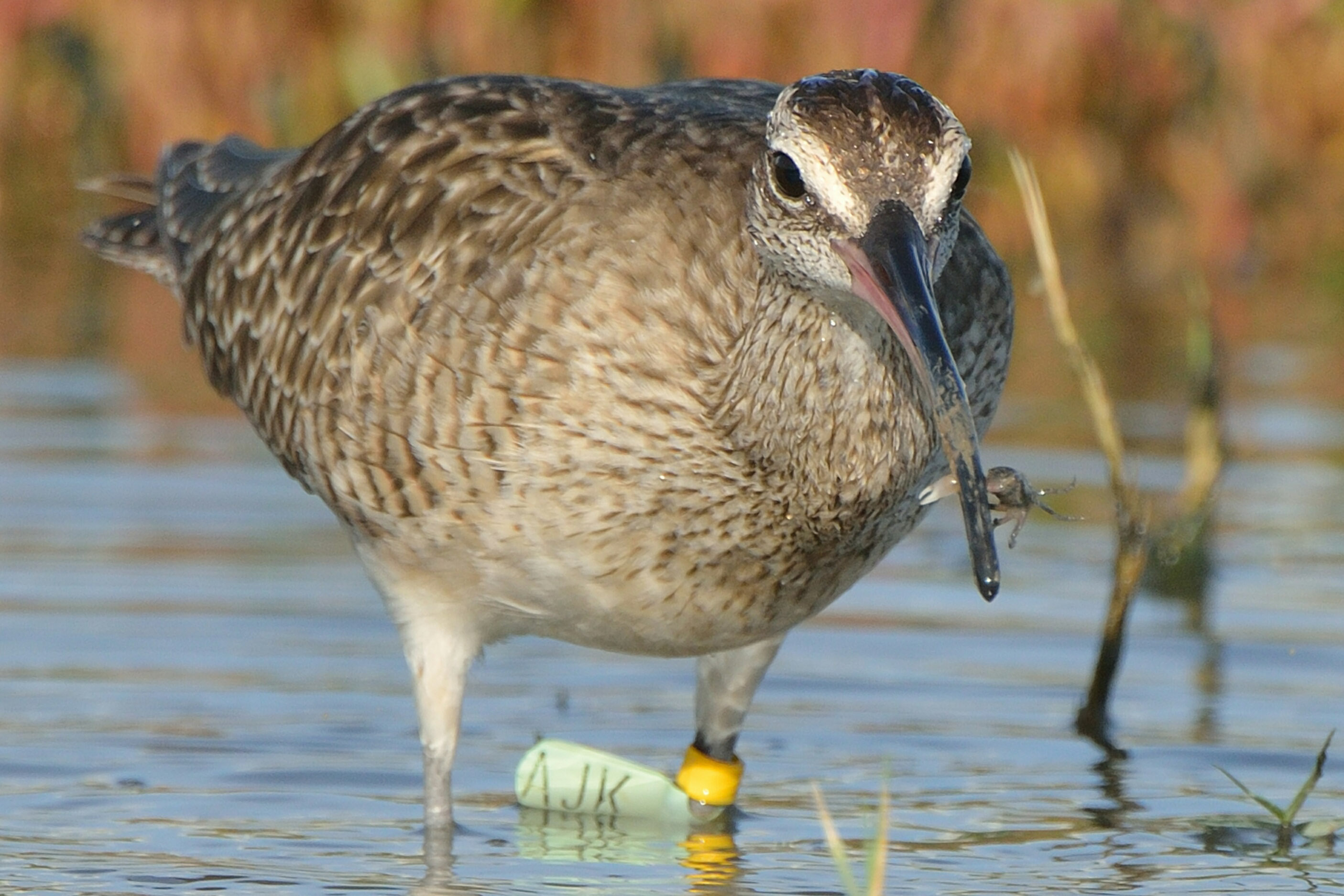In this horizontal, rectangular wildlife photograph, we see a close-up of a large, wading bird standing in shallow water. The bird boasts a strikingly long, dark brown beak and big, round body adorned with a mix of brown, black, and gray feathers. Its eyes are black, with a distinct white patterned region above them, and a black-colored forehead. The bird is wearing a yellow ankle bracelet with a silver tag embossed with "AJK" on one of its short legs. The surrounding water features some vegetation, and in the blurred background, we can make out trees with fall foliage and some sticks emerging from the water. The bird is holding what looks like a crab or a small water insect in its beak, adding a dynamic element to the serene outdoor scene.